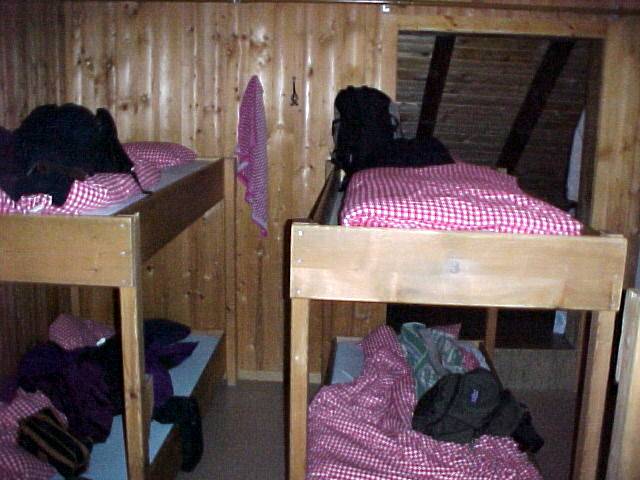The photo captures a rustic, night-time scene inside what appears to be the attic or upper level of a wooden cabin, illuminated by flash. The room features wood-paneled walls and various timber elements, giving it a cozy, yet basic feel. Four wooden bunk beds, arranged side by side in pairs, dominate the space. Each bunk is outfitted with red and white checkered bedding, reminiscent of a classic tablecloth pattern. The beds are unoccupied but appear lived-in, with rucksacks and personal items strewn across them, suggesting recent arrivals who have not yet settled in. Hanging on the back wall, a towel adds to the informal, utilitarian atmosphere. A window, possibly part of the cabin's slanted roof supported by metal braces, adds a slight outside view, completing the scene of an untidy yet welcoming woodsy retreat.